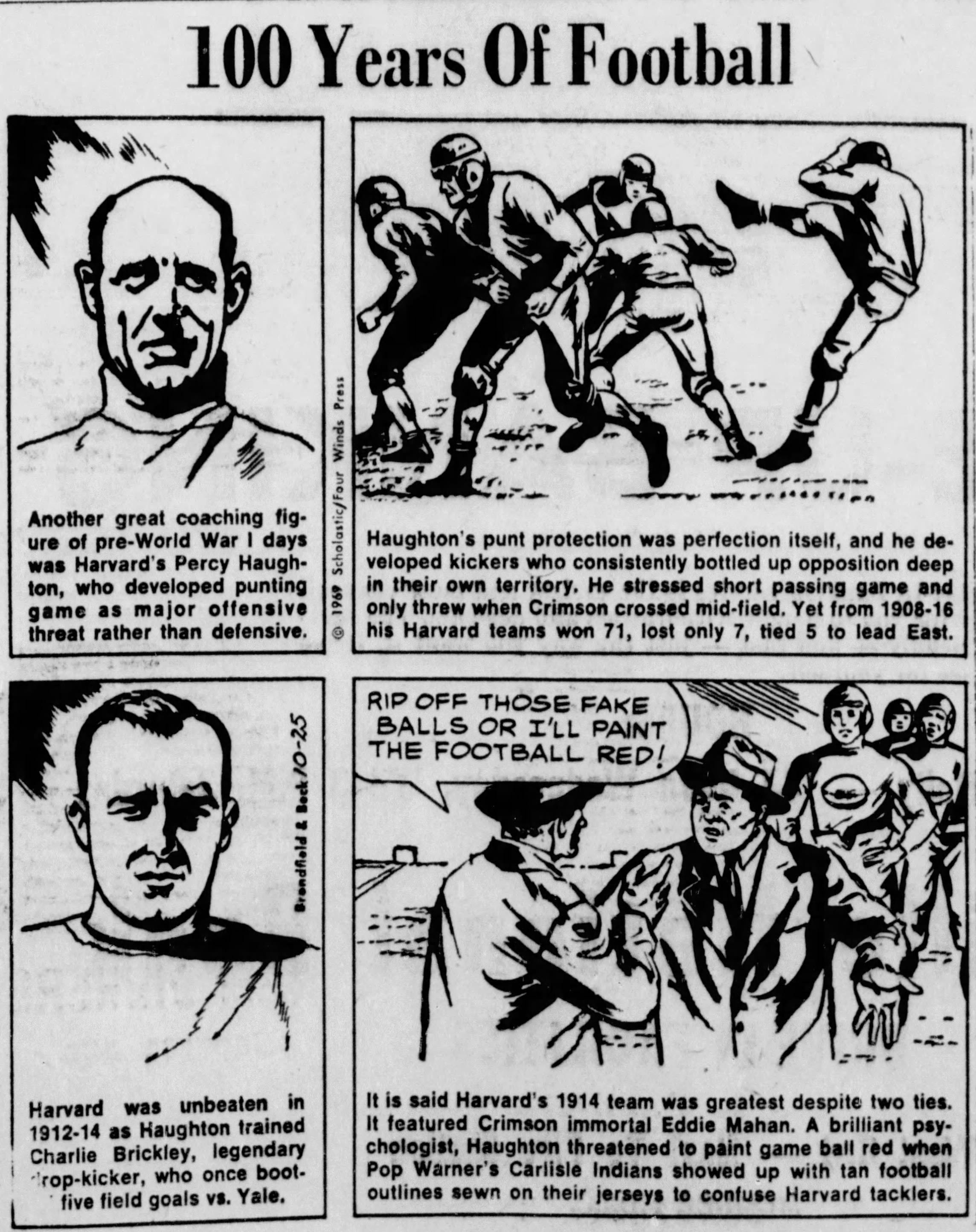The black-and-white cartoon, likely from a historical newspaper dated 1969, titled "100 Years of Football," features four distinct panels, resembling a comic or picture book page. The top left panel depicts Percy Houghton, Harvard's pre-World War I coach, who innovated by making punting an offensive strategy. Adjacent to this, the top right panel illustrates a group of football players, adorned with leather helmets, as part of Houghton’s punt protection unit designed to hinder opponents deep in their territory. The bottom left panel showcases Charlie Brakely, a legendary drop kicker who contributed to Harvard's unbeaten 1912 season. In the bottom right panel, two men in suits converse with football players in the background, with one expressing frustration over deceptive tactics by saying, "Rip off those fake balls or I'll paint the football red."